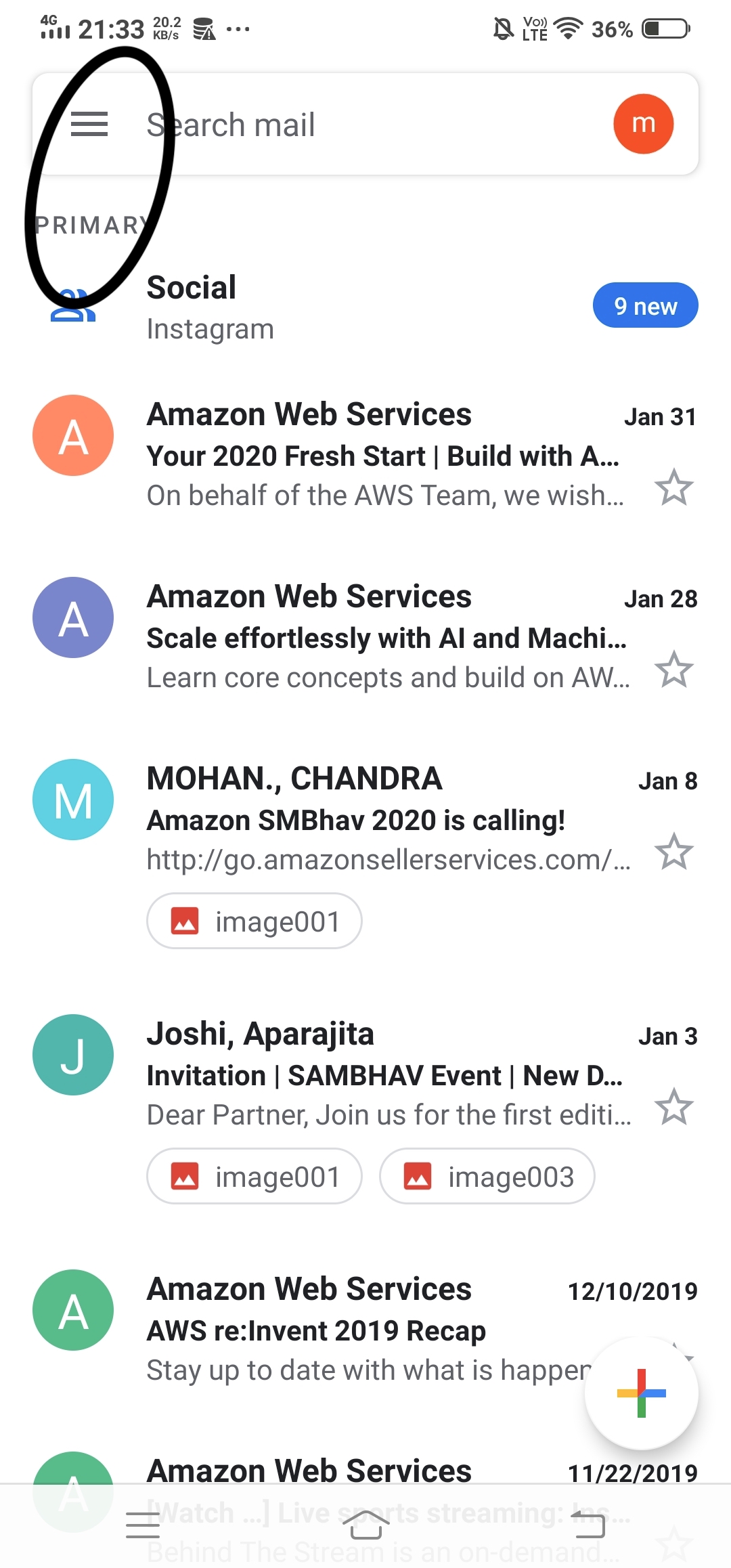**Detailed Caption:** 

The image showcases a white background with various UI elements that appear to belong to an email or communication interface. In the top-left corner, the battery percentage is displayed as 36%, next to the time which alternates between "21" and "23". Directly below, there is a search mailbox icon represented by three horizontal lines on the left and a red circle with an "M" in it on the right.

The central part of the image features a large black circle highlighting the three lines and the word "Primary." To the right of this section, there is a blue box with the label "9new."

Further below, there is a sequence of notifications:
1. A red circle with an “A” labeled "Amazon Web Services: Your 2020 Fresh Start" dated "January 31st" with a star.
2. A blue circle with an “A” labeled "Amazon Web Services: Scale effortlessly with AI and matching," dated "January 28th" with a star.
3. A light blue circle with an “M” labeled "Mohan Chandra: Amazon SMBhav 2020 is calling," dated "January 8th" with a star.

Also visible is a smaller white box with a red square containing white text that says "image 001" underneath it. This is followed by a darker blue box with a "J" that reads "Joshi Aparajita: Invitation to Sambhav event," dated "January 3rd" with a star. This particular notification includes two images denoted as "image 001" and "image 003".

Additional elements include:
- A green dot with an “A” labeled "Amazon Web Services: AWS re:Invent 2019 recap," dated "12-10-2019."
- A white circle with a colorful plus sign (red, green, blue, and yellow).
- A partially cut-off green circle with an “A” labeled "Amazon Web Services," dated "11-22-2019."

At the bottom of the image, there is a control bar with three lines, an upward arrow, and a semi-square.